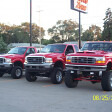The photograph is small, approximately 2x3 inches, capturing three solid red pickup trucks parked side-by-side on a paved lot that resembles a car dealership. A tall sign looms over the scene, although the illegible text makes the exact establishment unclear. The trucks, differing in sizes and grill designs, flaunt enormous black wheels and raised suspensions, revealing significant gaps between the rims and the wheel arches, with support bars visible beneath. Behind the trucks, power poles and trees punctuate the landscape, adding depth. Though one truck is identified as a Ford F-150, the exact makes of the others remain uncertain, with one speculated to be a Toyota. The photograph, possibly from a digital camera due to the partial date stamp ending in "625," hints at a possible connection to an Auto Zone, inferred from a faded sign in the background.